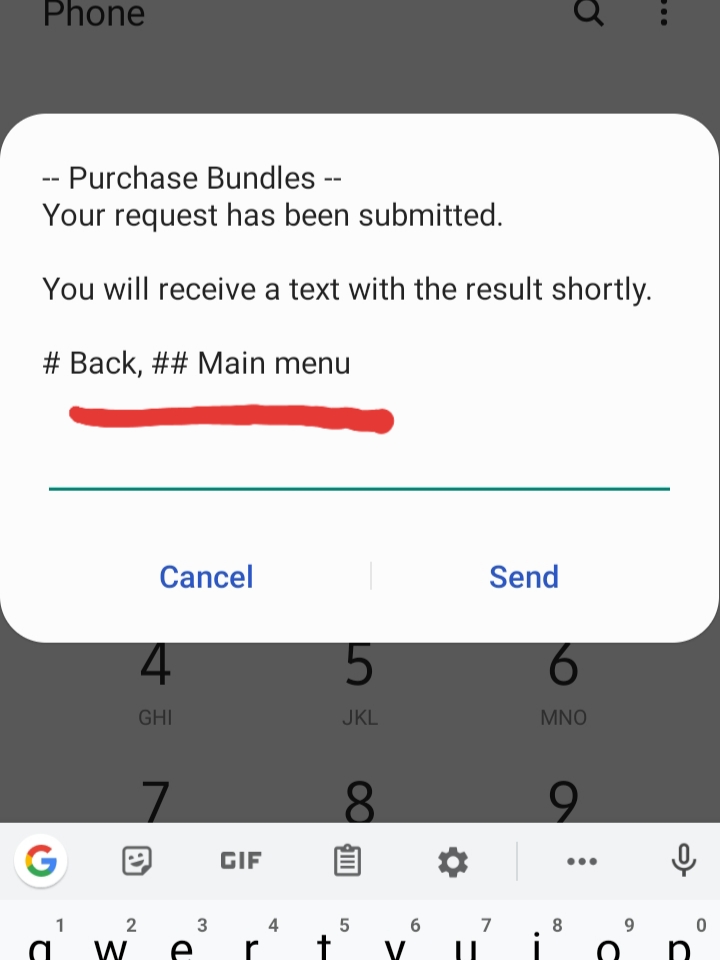This image captures a cell phone screenshot displaying a pop-up notification. The pop-up features a white background with black text stating, "Purchase Bundles -- Your request has been submitted. You will receive a text with this result shortly." The phrase "Hashtag Back Hashtag Hashtag Main Menu" is prominently underlined in red. Below this, a green line spans the width of the pop-up. There are two interactive links beneath the text: "Cancel" and "Send."

The background shows the cell phone’s number pad, which is slightly darkened by the overlay of the pop-up notification. At the bottom of the screen, the keyboard interface partially appears, offering quick access icons including a Google 'G,' a smiley face within a square, the word "GIF," a lined paper symbol, a settings cog, an ellipsis for additional options, and a microphone icon for voice input.